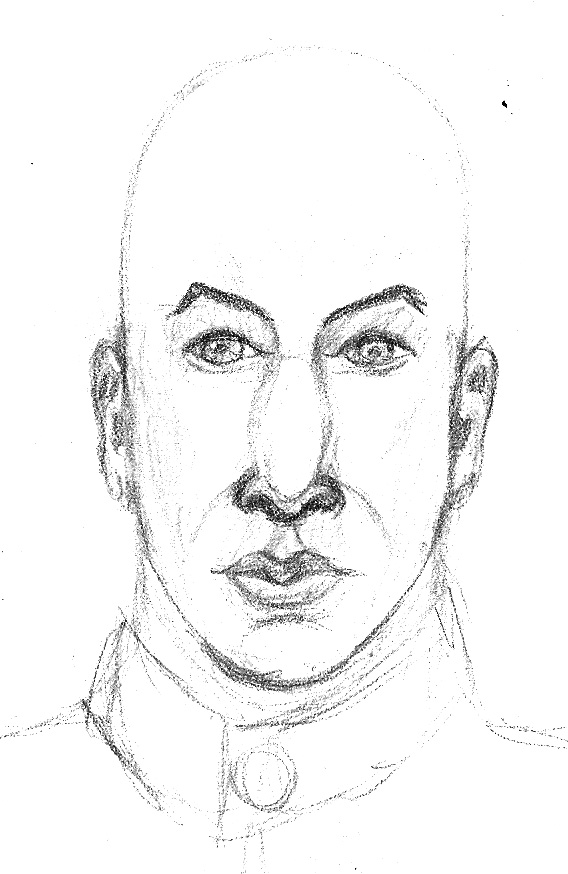This illustration is a meticulously hand-drawn portrait of a bald man with a focused and intense gaze, directed straight at the viewer. It appears digitally scanned, evident from the visible pencil sketch marks and tiny gaps where the pencil dragged on the paper. The drawing captures the nuances of the man's face and upper shoulders, outlined with careful pencil strokes and subtle shading that convey a 3D effect.

The man is dressed in a high-collared, buttoned storm jacket, hinting at a military or formal appearance. His strong eyebrows, almost black in color, frame his eyes, which are shaded with varying intensities, making the right pupil slightly lighter. His nostrils are prominently shaded in black, emphasizing the contours of his wide nose. His lips are pursed, with the top lip rendered in dark gray and the bottom lip in a lighter shade, enhancing the depth and realism.

The sketch employs multiple lines, especially around the neck and collar, to build detail and dimension, contrasting with the single line around the bald head. The man’s ears are large yet proportionate to his face, contributing to the overall lifelike quality of the portrait. The illustration is entirely monochromatic, relying on the mastery of pencil shading and line work to create a striking and detailed representation of the man.